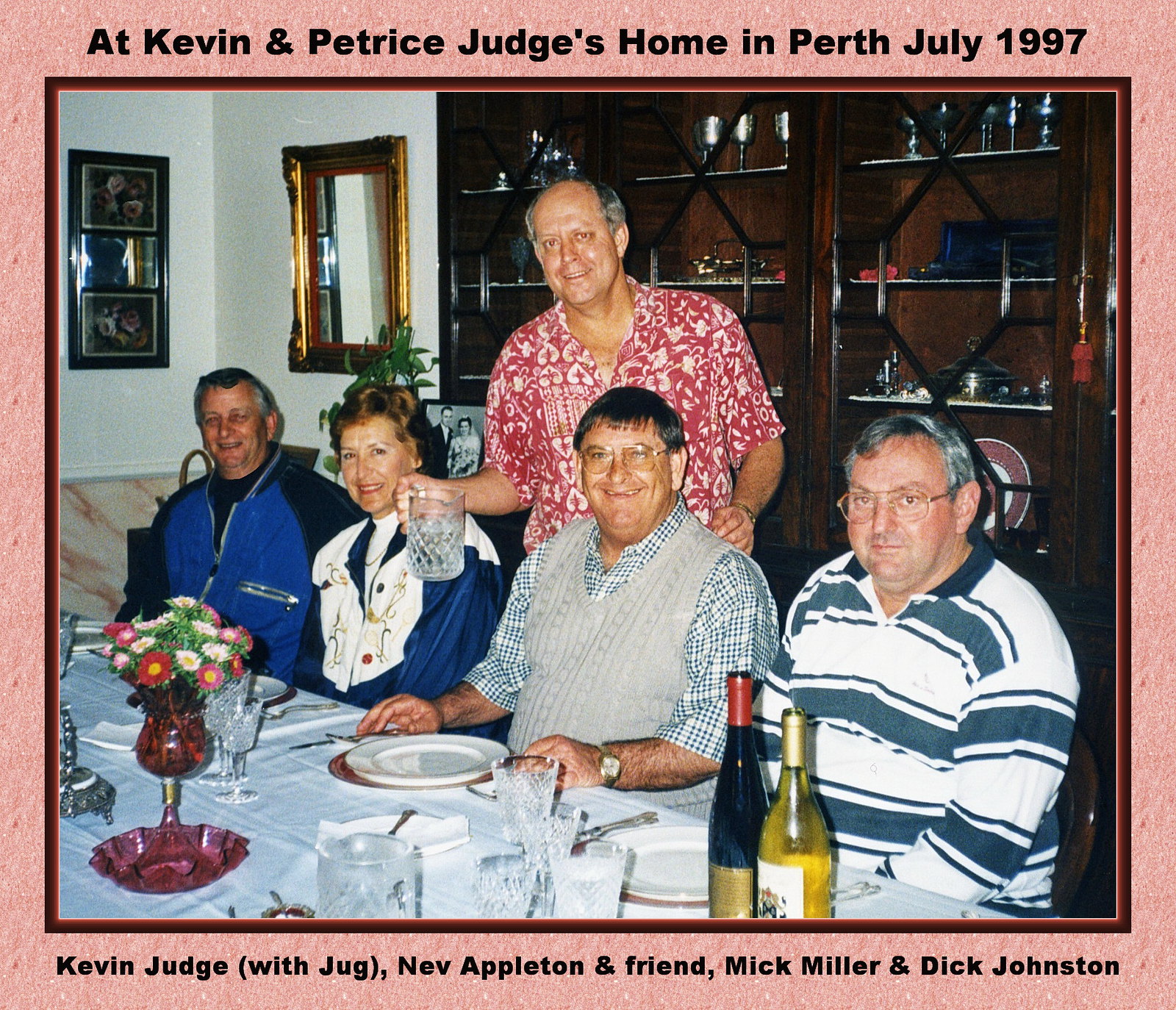The image depicts a family gathering at Kevin and Patrice Judge's home in Perth, July 1997. The photo is bordered with a light pink frame, bearing text at the top and bottom. The dining scene shows four men and one woman, sitting at a table in a well-decorated dining room. Kevin Judge, holding a jug, stands between a female and another male, pouring water into the glasses on the table. Nev Appleton, Mick Miller, and Dick Johnston are also present, sitting around the table covered with a white tablecloth. The table is elegantly set with white china and numerous crystal wine glasses, complemented by two wine bottles and an assortment of colorful flowers at the center, including red, white, yellow, and purple blooms. Behind them, a cherry-finished china cabinet and a gold-framed mirror enhance the room's decor. The white walls host several pictures, adding to the homely ambiance of this indoor, mid-day gathering.